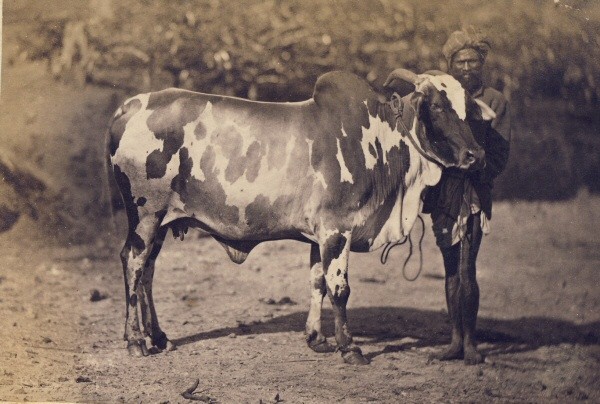This is a vintage, possibly sepia-toned photograph, now yellowed with age, showing a Middle Eastern man and a large, spotted cow standing on a sandy, dirt landscape. The man, with a bushy beard and a headdress, is dressed in layered dark clothing, including what appears to be a jacket over a shirt or tunic ending at his thighs. His feet seem to be bare. He stands beside the cow, which has a prominent bulge on the back of its neck and one visible horn. They both face the camera, with the cow's head oriented to the right of the picture and its body extending towards the left. In the background, there seems to be some vegetation, possibly plants or a pond, casting shadows on the ground.